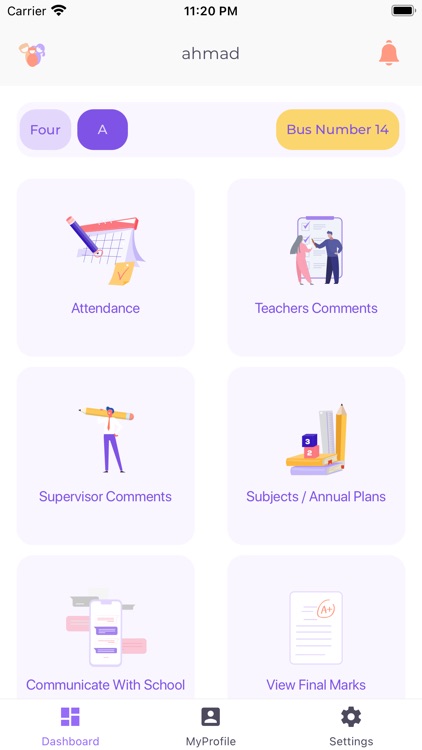**Caption:**

The screenshot appears to be from a mobile device, depicting the interface of an educational or school management app. It's 11:20 PM as indicated by the clock in the top right-hand corner, alongside battery and Wi-Fi icons showing the device's connectivity status. 

At the very top, a bell icon and another symbol accompany the name "Ahmaud." Below are various bullet points, set against blue and gray backgrounds, detailing important information: "4A, bus number 14." 

Columns of icons follow, each representing different sections of the application:

1. A calendar icon with a pencil, labeled "Attendance."
2. "Teacher Comments," illustrated by an image of a woman in a pink dress and a man in a long-sleeved shirt with dark slacks beside her.
3. An icon for "Supervisor Comments" showing a man adorned in a white shirt, red tie, and blue pants, with a pencil near his face.
4. "Subjects/Annual Plans," depicted by books stacked high with a pencil vertical among them.
5. "Communicate with School."
6. "View Final Marks."

Additionally, there are icons for accessing the "Dashboard," viewing "My Profile," and adjusting "Settings." Each section appears to be easily navigable and tailored to provide thorough information and interaction options for students and parents.